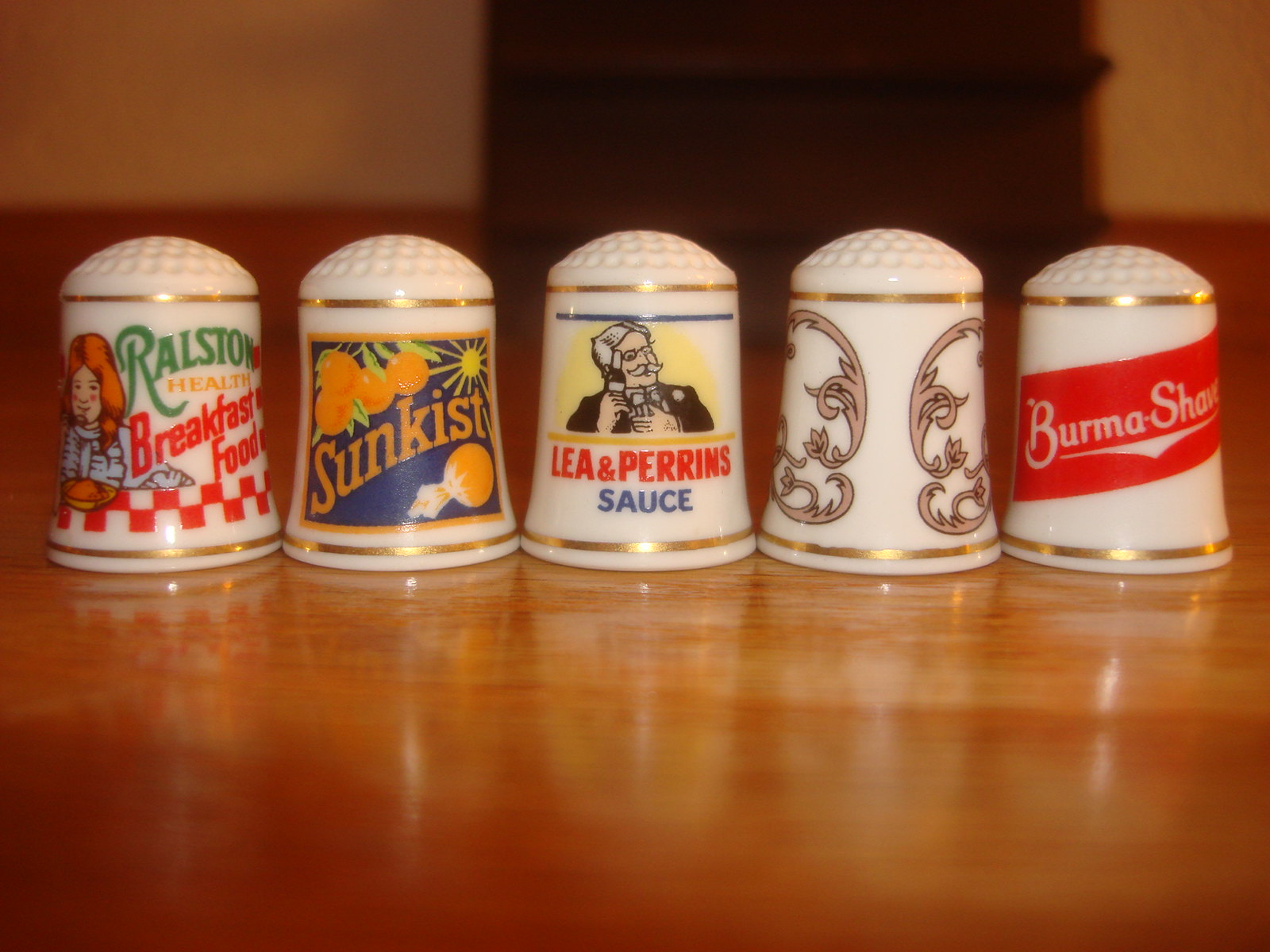The image displays five short and wide decorated salt shakers arranged in a row on a highly reflective, shiny wooden surface. Each shaker, predominantly white, showcases a distinct retro design. 

The first shaker features the words "Ralston's Breakfast Foods" alongside an old-fashioned illustration of a girl with orange hair and red blush holding a dish. Following that, the second shaker depicts a vibrant blue background with a bright sun, four oranges, and a lemon, bearing the text "Sun Kissed." 

In the center, the third shaker advertises "Leigh and Perrins Sauce" and includes an image of an old-fashioned man in a powdered wig. Next to this is the fourth shaker, adorned with a simple brown paisley pattern.

Finally, the fifth shaker sports a bold design with red and white stripes and the phrase "Burma Shave" prominently displayed.